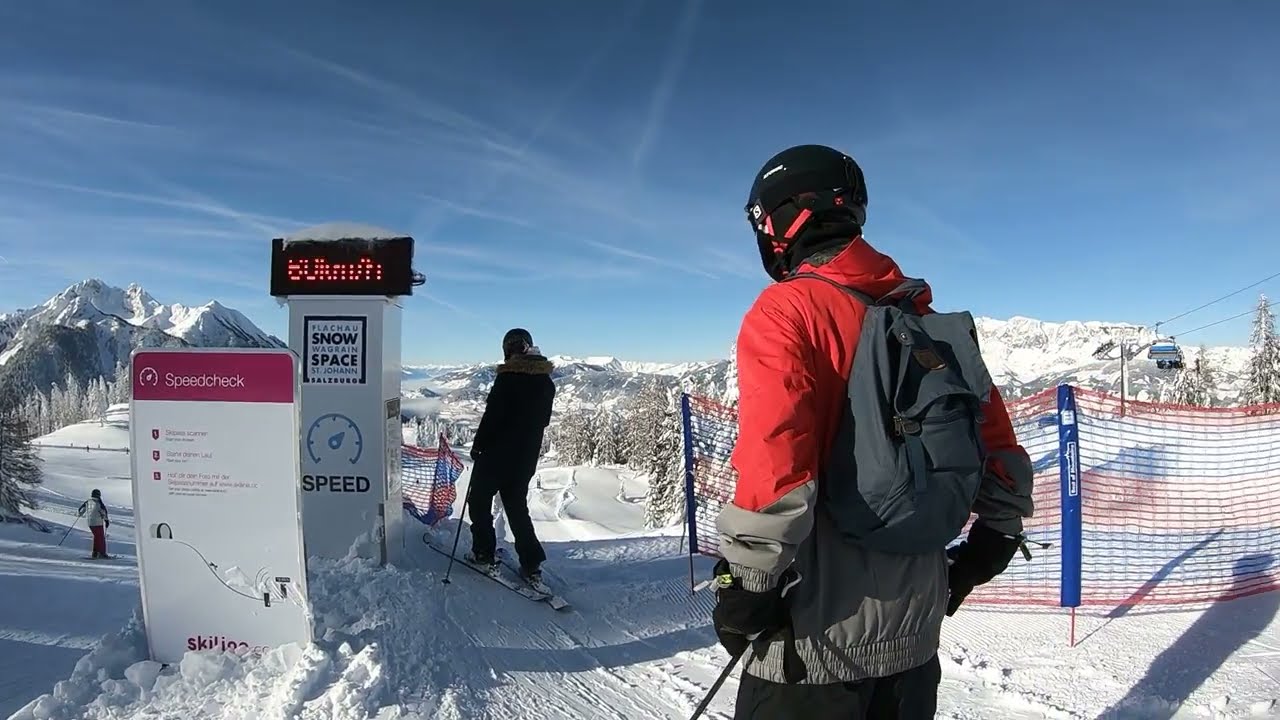In this photograph, several people are preparing to ski on a snow-covered slope. There are about three individuals clearly visible, all equipped with full skiing gear, helmets, and standing near a maroon-background sign that reads "Speed Check" in white letters. Just behind this sign, there's another display indication showing speed with yellow lights. To the right, there's a red plastic guide fence on poles. The skiers, positioned centrally in the image, appear to be waiting in line to descend a steep slope. The backdrop features snow-covered trees, distant mountains, and a ski lift. Various colors populate the scene, including white, red, black, orange, gray, tan, blue, and turquoise, highlighting the diverse skiing attire and natural surroundings. The sky is mostly clear with minimal clouds, emphasizing the outdoor, snowy day setting.